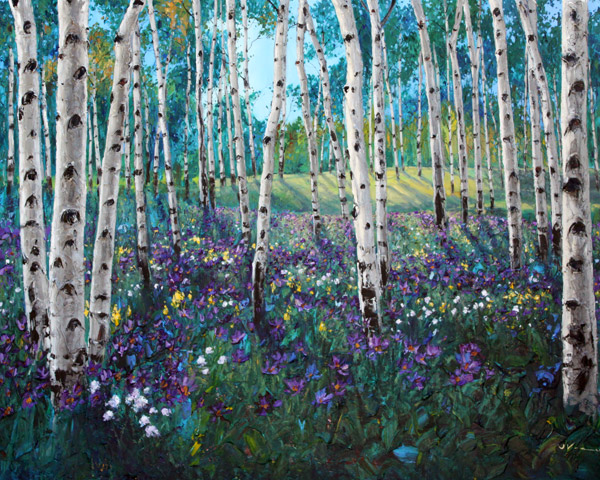This image, likely a painterly interpretation rather than a photograph, captures a vibrant, natural landscape marked predominantly by green hues from grass and various plants. At the bottom, a lush carpet of flowers unfolds, showcasing a rich palette of mostly purple and blue blossoms, with accents of yellow, white, and light pink. Slender tree trunks, numbering at least a couple dozen, stand among the flowers. These trunks are predominantly white with occasional black spots, resembling birch or aspen trees. The image is vertically oriented, hinting at a daytime setting as patches of blue sky and white clouds peek through the leafy canopy at the top. In the composition's background, the density of trees decreases, opening up to reveal more green space before the tree cover thickens once more. Overall, the scene feels almost like an outdoor cathedral, with the trees forming a natural circle, creating a serene, enclosed grassy patch at the center.